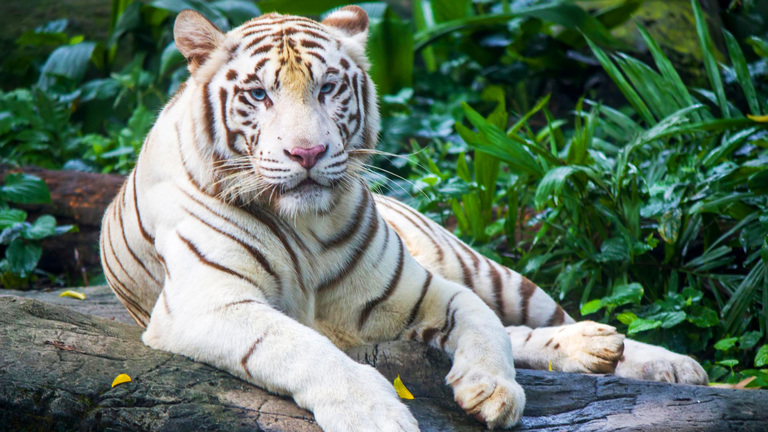The photograph captures a white tiger with subtle orange-beige hues in its predominantly light-colored fur and distinct black stripes. The tiger is resting majestically on a fallen tree branch, positioned up slightly to the left of the image center. Its captivating blue eyes are fixed on the photographer, with its mouth slightly open, revealing no teeth. The scene is set outdoors, within a lush, green enclosure likely in a zoo. Surrounding the tiger are small plants, grass, fallen leaves, and various shades of greenery, all under an overcast or humid, rainy atmosphere, creating a natural yet slightly blurred backdrop.